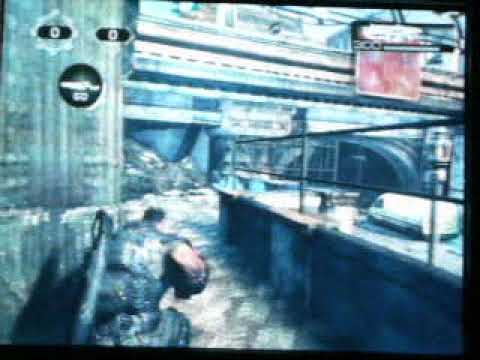This screenshot captures an immersive moment from a third-person shooter video game, widely agreed to be either "Resident Evil 5" or "Gears of War," showcasing an environment that evokes a sense of familiarity and nostalgia. The image is characterized by a blurry, washed-out effect that gives it a slightly older and foggy appearance. Dominating the foreground is a very bulky soldier character in a crouched posture, positioned approximately four feet from the elevated camera, which hovers just above his head. The soldier is partially concealed behind a large stone pillar to his left, peering into a futuristic courtyard area of a city with green and blue hues. The courtyard features a raised platform, likely designed for a train, running horizontally across the scene with arches beneath it. The character, seemingly in cover and holding a gun with another on his back, is ready for impending action in an environment scattered with elements like gates, railings, and potentially rubble, suggesting a tense and tactical scenario.